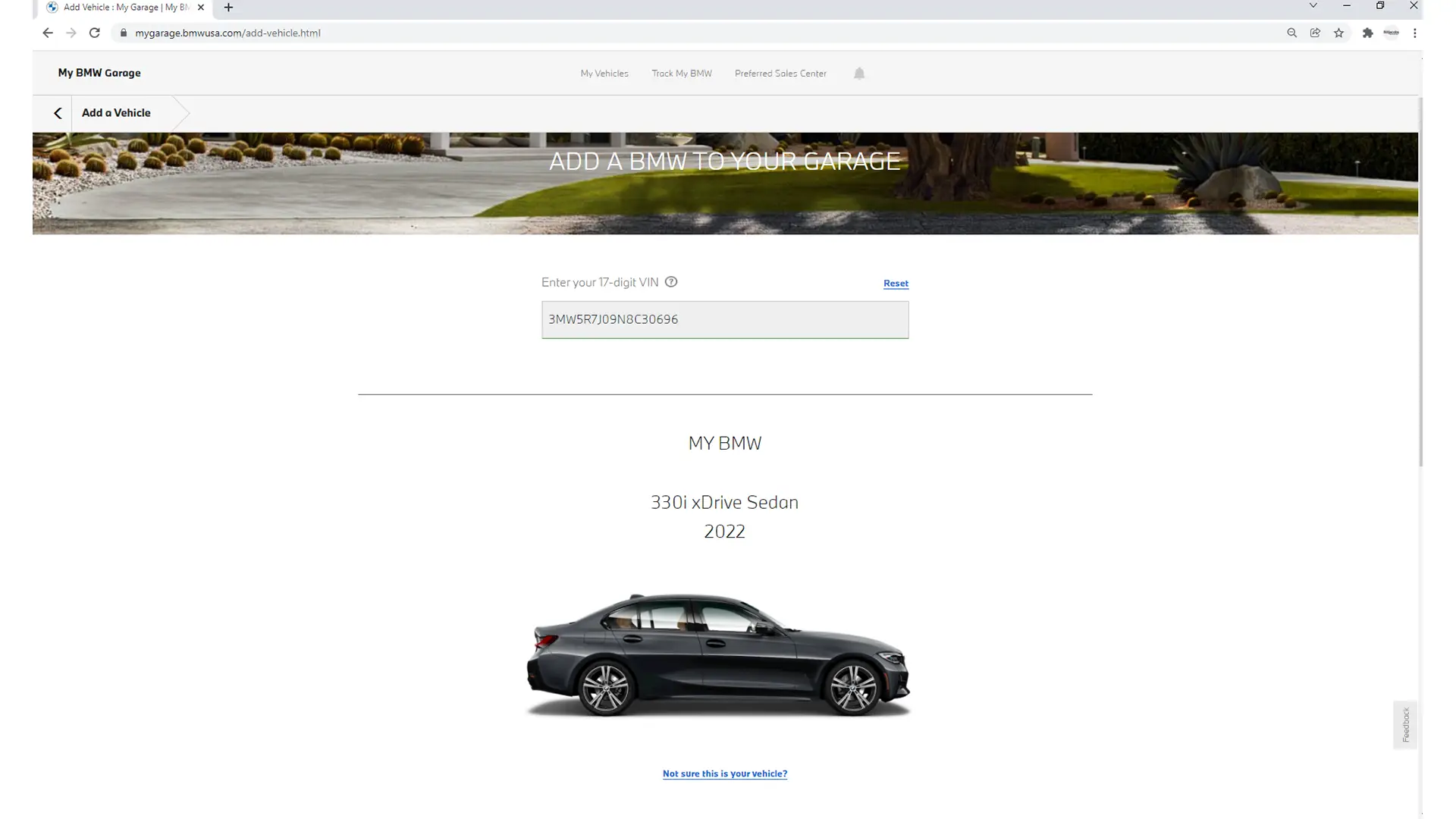The screenshot appears to be of a website, likely BMW USA, specifically a section called "My BMW Garage." At the top of the page, the URL confirms it's from BMW USA. The header of the page is labeled "Add a Vehicle." 

Below the header, there's a banner displaying an image of a BMW with a prompt to "Add a BMW to Your Garage." Following the banner, there is a form inviting users to enter the 17-digit VIN number of their BMW, with an accompanying "Next" button for submitting the information.

Further down the page, there is an image of a 2022 BMW 330i xDrive Sedan in a dark, charcoal gray or black color, shown from a side angle, facing to the right. Beneath this image, there is a text prompt asking, "Not sure this is your vehicle?" suggesting that the purpose of this section is to verify the user's BMW model rather than solely adding a new vehicle to the virtual garage.